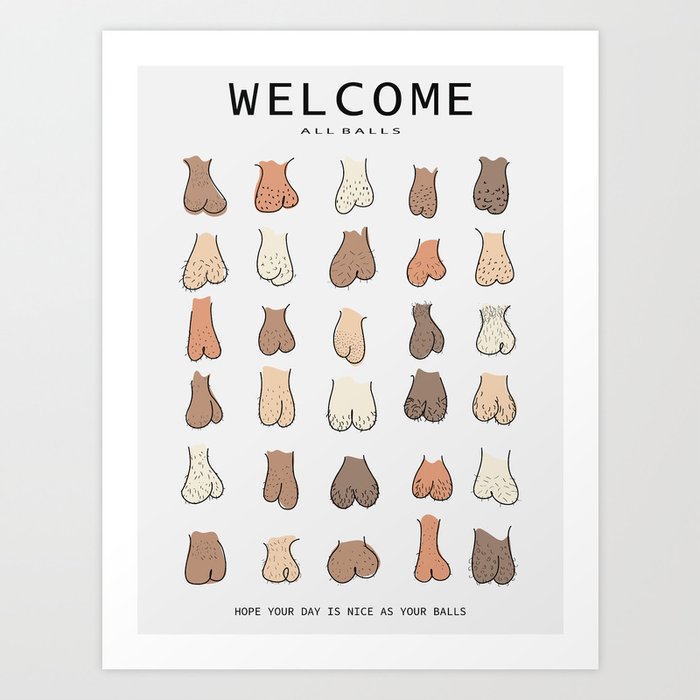The image features a poster with a thick white border and a background in a light blue-gray hue, slightly lighter than the outer background. Dominating the top of the poster, in large, bold black capital letters, is the word "WELCOME." Just below this, in smaller black capital letters, is the phrase "ALL BALLS." The central part of the poster is filled with illustrations of various cartoon-style balls arranged neatly in six rows of five columns, totaling 30 balls. These balls vary in color—ranging from dark brown to light peach—and in texture, with some depicted as hairy and others smooth. The artistic style suggests they are hand-drawn. At the very bottom of the page, in small black print, the poster cheekily reads, "HOPE YOUR DAY IS NICE, AS YOUR BALLS." The overall composition hints at a humorous take on personal grooming, particularly emphasizing male hygiene.